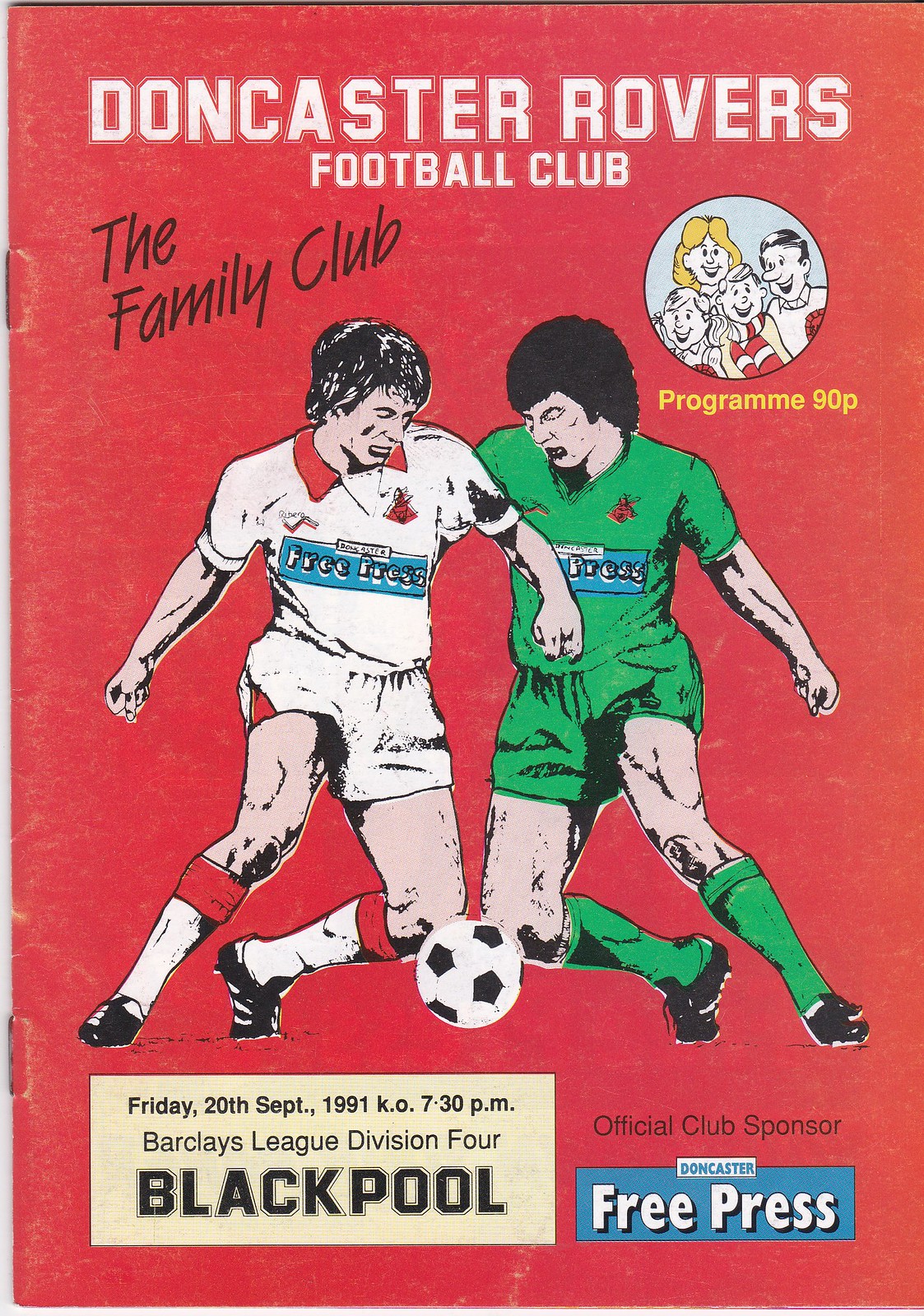The cover of a soccer magazine from 1991 features a vibrant red background centered around a colorful illustration of two soccer players in the heat of the game. The player on the left dons a white uniform with a red collar, while his opponent on the right wears green. Both players have the words "Free Press" emblazoned across their chests, and they appear to be contending for the ball at their knees. Above them, the title "Doncaster Rovers Football Club" is prominently displayed in white letters. On the upper left, the text "The Family Club" is written in black, accompanied by a circular illustration to the right depicting a smiling family of four. Below this, a yellow box reads "Program 90P." Further down, a creamy yellow rectangle provides details about the event: "Friday, 20th September 1991, KO, 7.30pm, Barclays League Division 4, Blackpool." To the right of this, in smaller black text, it states "Official Club Sponsor." At the bottom right, a blue rectangle includes the white text "Doncaster Free Press." The cover exhibits signs of wear with noticeable scratches and scuffs, reflecting its age and historical value.